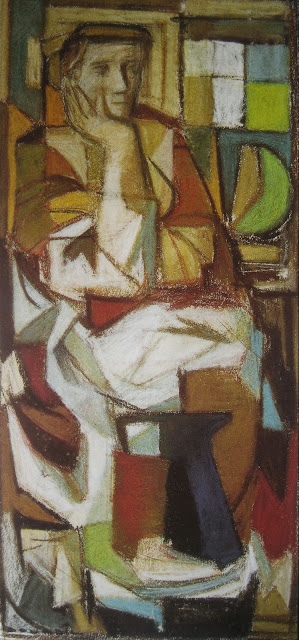This vertically rectangular, abstract artwork, rendered in pastel oil colors, depicts a young Caucasian man sitting contemplatively with his right hand under his chin, reminiscent of Rodin's The Thinker. The geometric, surreal style features multiple squares and angular shapes, predominantly in earth tones such as white, red, mustard, and lime green. The man is dressed in a long-sleeved tunic with red and white detailing, suggesting a robe. He has red hair and a pointed face, with fair skin and a notably thick right forearm. The background includes a square window with colors of white, mustard, and lime green, positioned over his left shoulder. To his left, which is the right side of the image, there is a large round object and a door directly behind him. At his feet, partially entwined in the robe, lies a dark blue or black pitcher. Scattered around him are objects resembling papers, a bucket, and an anvil, integrated into the composition with shapes like triangles and rhombuses. Overall, the colors include hues of red, green, gold, brown, yellow, and gray, creating a muted and cohesive palette.